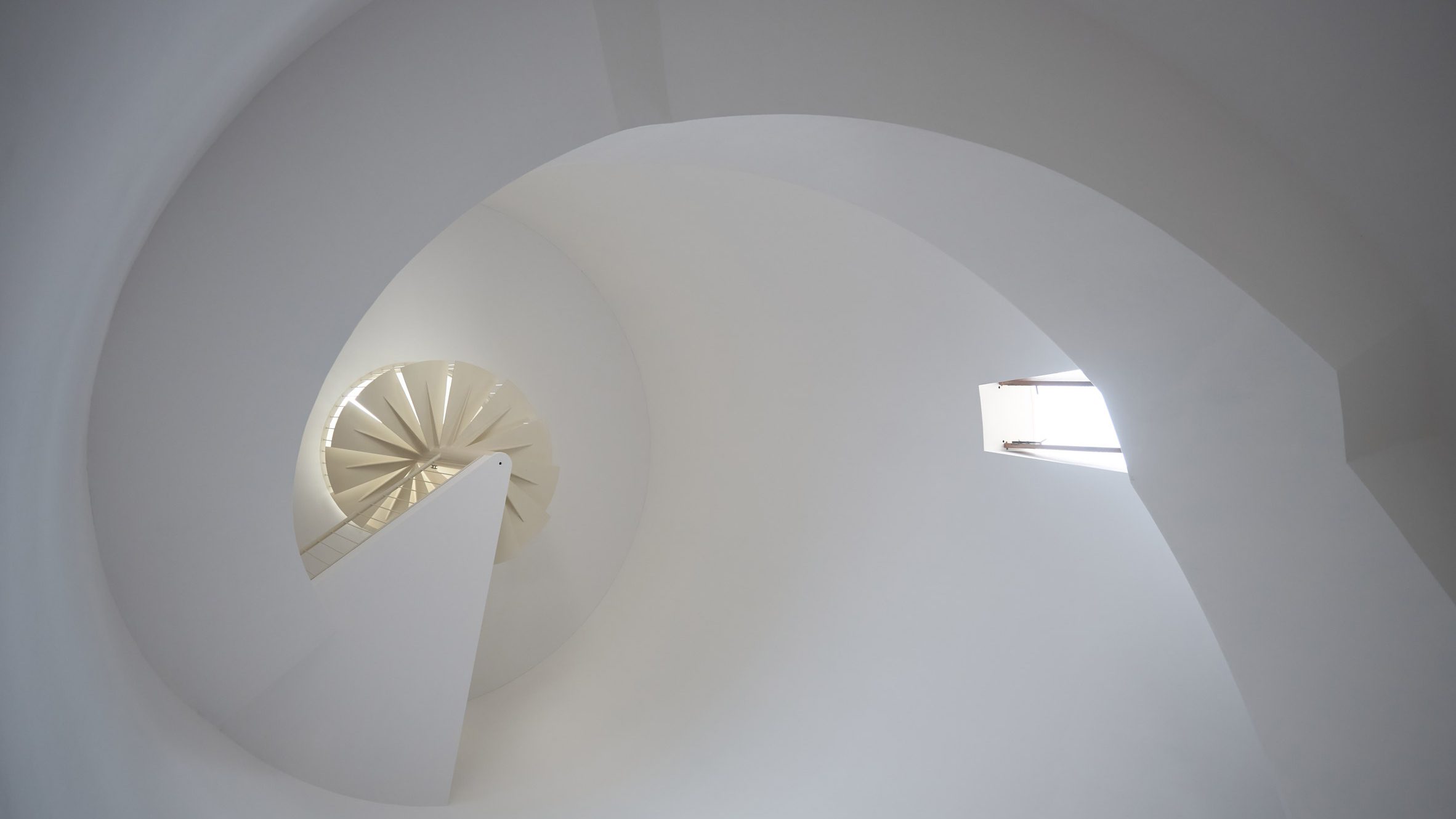The image depicts the interior of a building bathed in stark white tones. Dominating the upper section of the frame is an arching ceiling culminating in a triangular point, accented by a single grayish stripe along its curve. Centrally located on the left side is a circular structure resembling a fan, featuring a star-shaped design at its core. This fan-like object is cream-colored and nestled against the ceiling. Adjacent to this, towards the center-right of the photo, is a rectangular or triangular window, intersected by two horizontal bars, allowing light to stream through. The scene is framed from a low angle, enhancing the perception of height and curvature, reminiscent of a stairwell's winding form. The top right of the image appears slightly darker, adding depth and contrast to the bright surroundings.